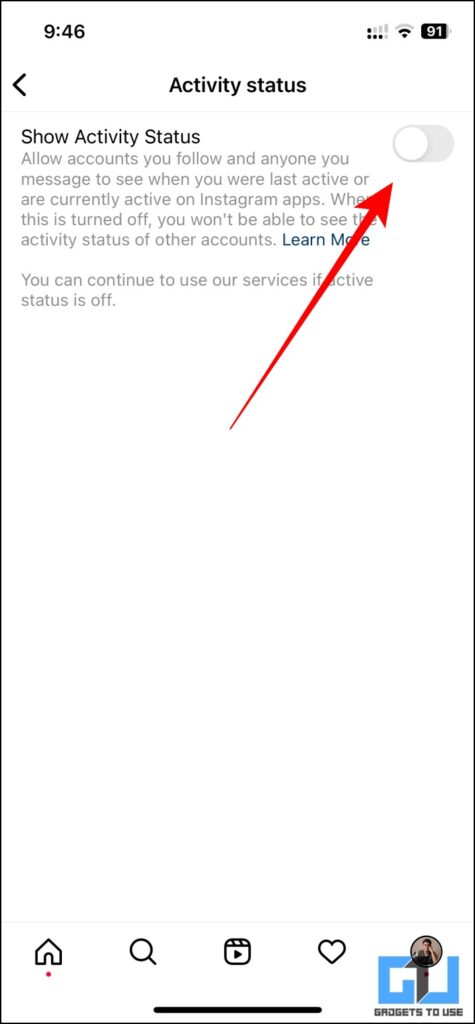The image is a screenshot of an Instagram settings page, specifically focusing on the "Activity Status" section. At the top, centrally aligned, is the header "Activity Status." Below this, to the left, is the option "Show Activity Status," accompanied by a toggle switch that users can turn on or off. A descriptive paragraph explains that enabling this feature allows accounts you follow and anyone you message to see your activity status on Instagram apps, whether you are currently active or were recently active. It also notes that if this feature is turned off, you will not be able to view the activity status of other accounts. Additionally, there is a "Learn More" link provided for further information. A distinctive red arrow points upwards towards the toggle switch, highlighting its location and functionality.